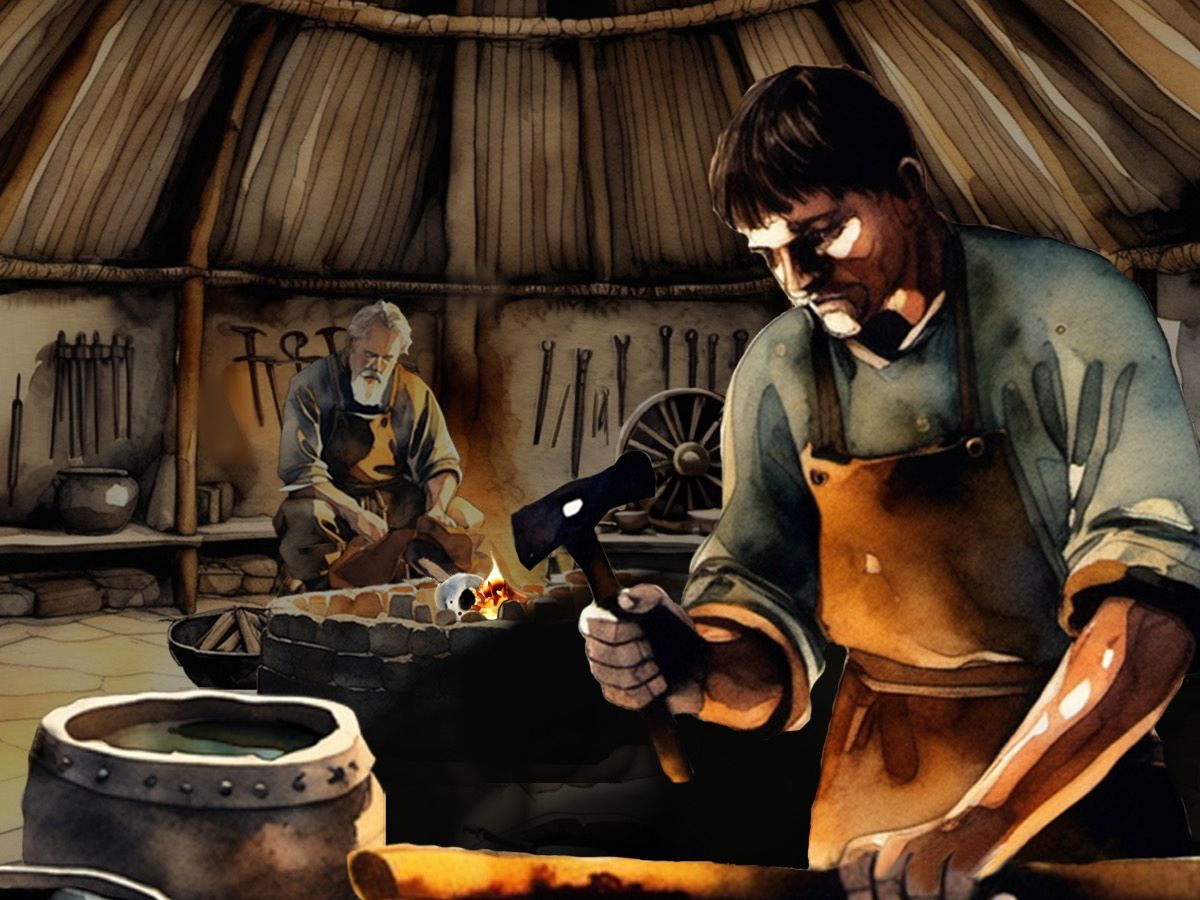The image is a detailed painting set in a dimly lit, rustic workshop resembling a blacksmith's hut. The hut, built from wooden poles and light brown timber, features gray stone walls adorned with various blacksmith tools including metal pliers, steel cutters, and a wagon wheel. The interior shows a light brown stone floor and a stone fire pit glowing with orange fire. 

In the background, an older blacksmith with gray hair, a white beard, and a mustache, sits at the fire pit, which he pumps with a brown device to feed oxygen to the flames. He wears a brown leather apron over a rolled-up shirt and gray pants. His task appears to involve heating a silver object in the fire. 

In the foreground, a younger blacksmith with short dark brown hair and bangs, dressed in a brown leather vest over a light blue shirt, hammers a piece of metal on an anvil. He grips the hammer in his right hand while steadying the metal with his left. Next to him is a cauldron likely used for cooling forged items. The overall scene exudes a sense of traditional craftsmanship, with the warm firelight contrasting against the cool tones of the tools and stone.